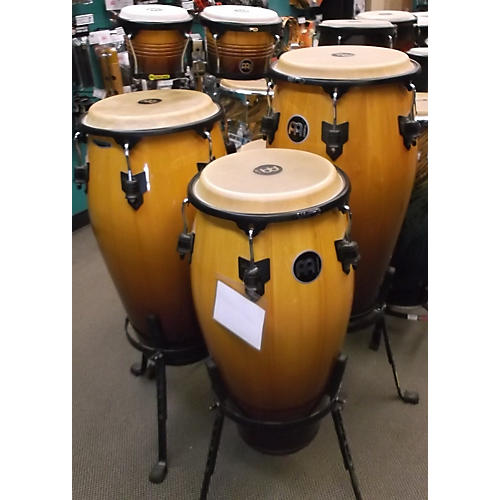The image depicts a room with a brownish-gray tiled floor, possibly a music store or a storage room. Central to the scene is a collection of tall, cylindrical drums. The foremost drum is light brown with a beige top encircled by a black ring, standing on a black stand with four legs. A white plastic tag hangs from this drum. Two additional drums are positioned behind it to the left and right, also light brown with black legs and beige tops, featuring black symbols or gadgets. In the background, more drums are visible, each varying slightly in shape and size. Some of the further drums are darker in color with striped, ridged exteriors, unlike the smoother surface of the drums at the front. The room's grayish-brown tile and green wall form the backdrop, adding contrast to the arrangement of drums. The setting is nondescript beyond these elements, focusing attention on the numerous drums arranged at different depths in the room.